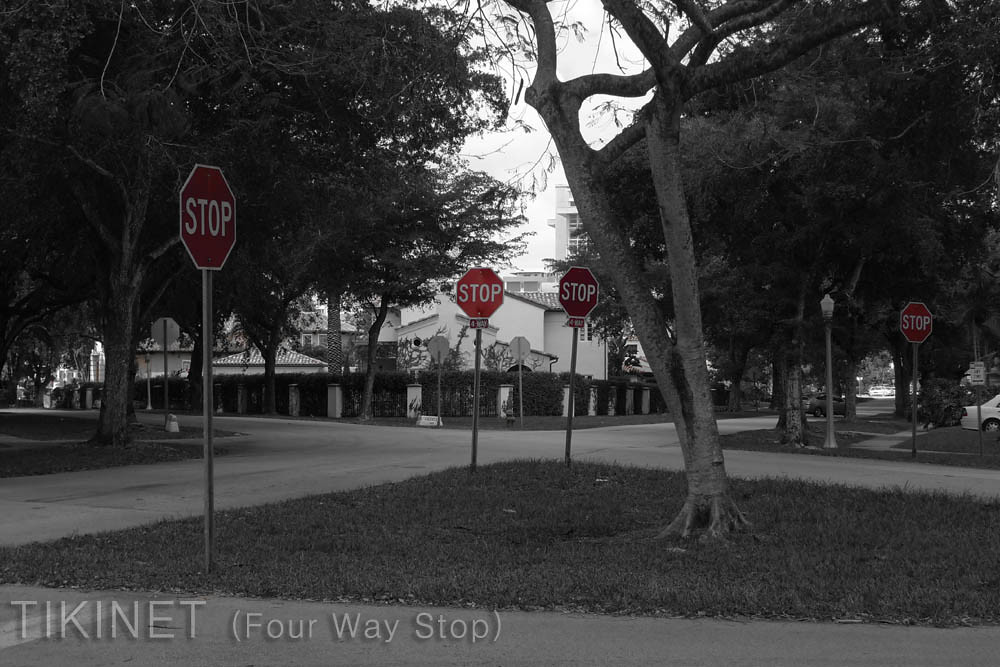This detailed black-and-white photograph captures an urban intersection area with vivid highlights. The focal point consists of multiple stop signs, notably colourised in red, creating a striking contrast against the monochrome backdrop. The signs are arranged in a sequence from left to right, with the leftmost sign positioned closest to the viewer. In the middle of the photograph, two stop signs border a square patch of lawn, which also contains a prominent large tree trunk curving into branches that blend with the sky. To the right, another stop sign is situated underneath a tree, adjacent to what appears to be a four-way stop intersection.

Near the bottom left corner of the image, translucent white text reads “Tinkernet, (four-way stop).” The intersection beyond the lawn features a commercial building with a white roof and supporting pillars. Flanking the building, two substantial trees frame a view of the sky. To the foreground right, a light post stands near the partial view of a white car's rear end. Additional visual elements include several trees scattered throughout the area, a backdrop of buildings, fences, and bushes, contributing to the urban landscape.